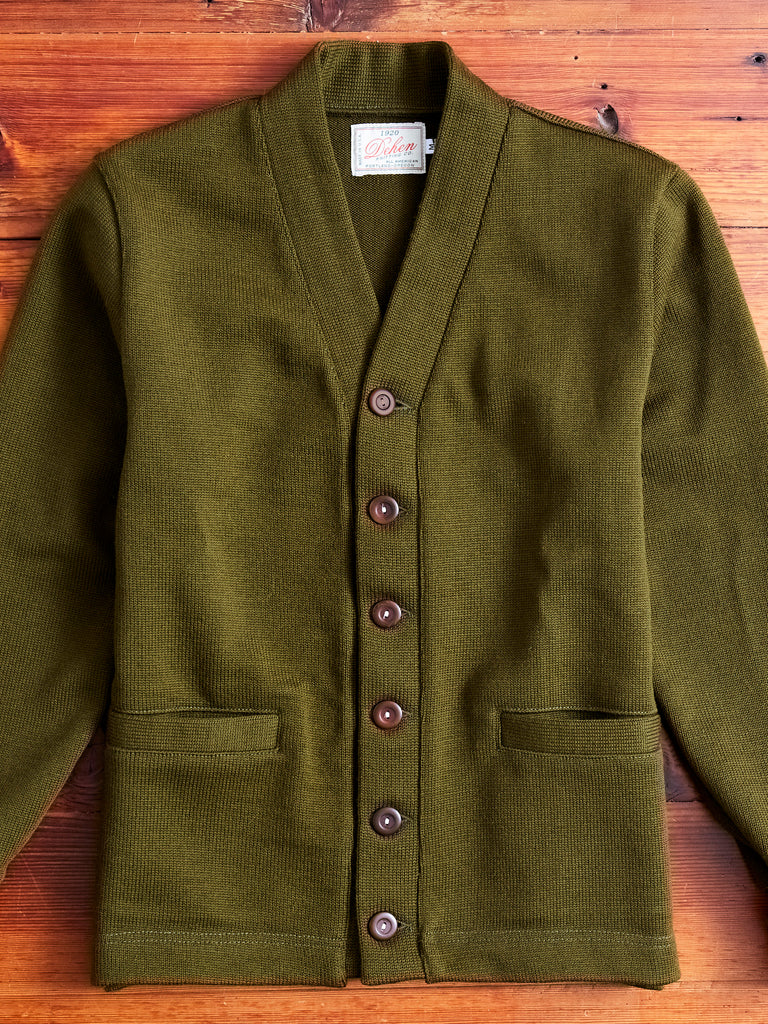This photograph captures a classic men's cardigan sweater laid out on a rich, warm brown wooden surface with visible knots, resembling a table or floor. The sweater presents a deep olive green, almost tobacco hue and is fashioned from a thick knit material. It features a V-neck design with a pronounced, thick collar leading into a button-down front, adorned with six round, brown buttons. The sweater includes two front pockets located near the hips with horizontal openings. The sleeves are partially visible, spread to the sides. There is a white rectangular label sewn into the back neck area, marked with red script that reads "Bowdoin," accompanied by a smaller tag indicating the size "M" for medium. The garment exudes a traditional style, reflecting a timeless appeal that might not be prevalent among younger generations today.